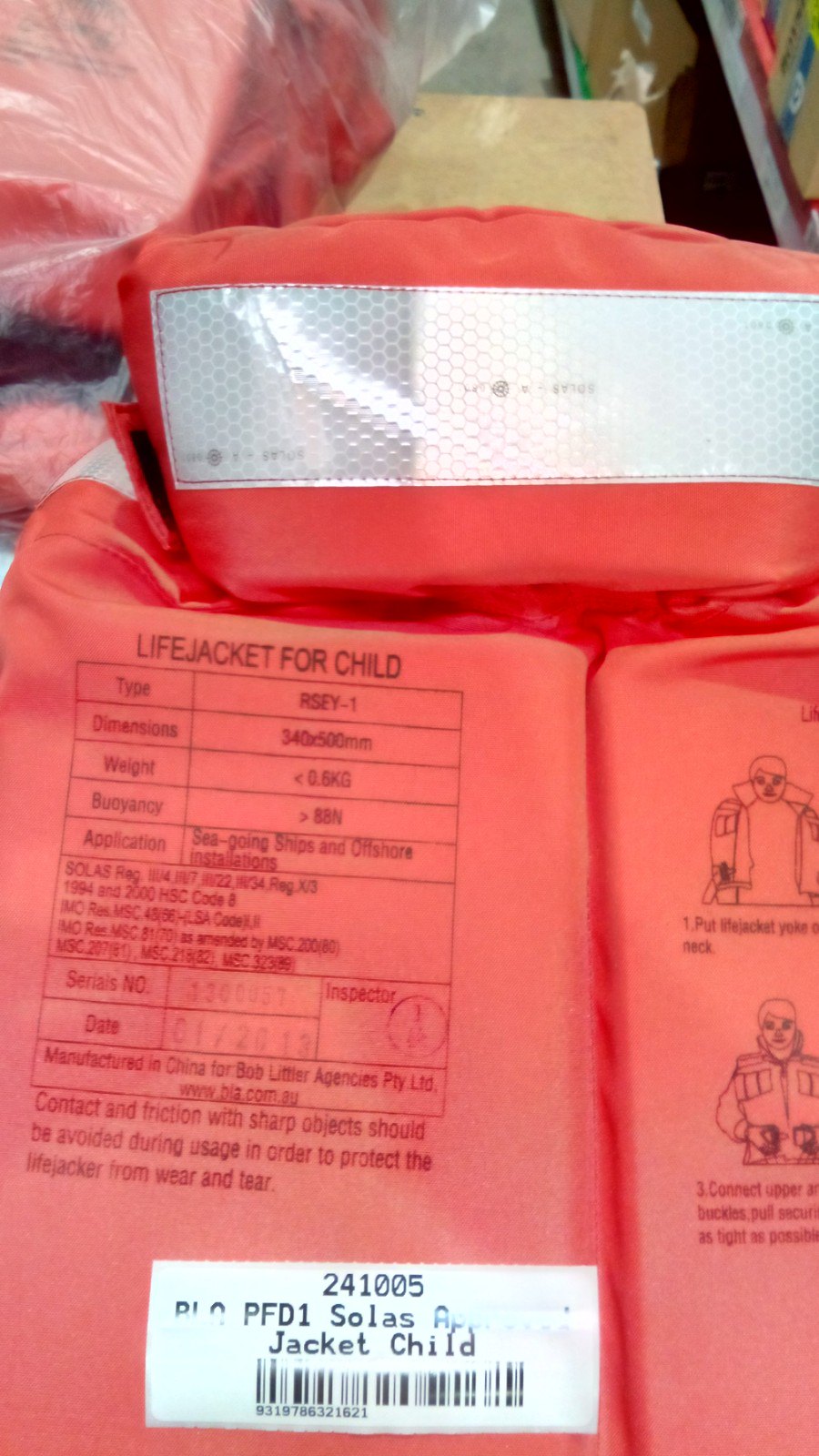This detailed photograph depicts a child’s life jacket in a store setting, captured in a close-up shot. The life jacket is an orange-ish red color with a reflective silver strip running across the top, designed for visibility and safety. Prominently displayed on the life jacket are several specifications and instructions. The text in black reads "Life Jacket for Child," along with additional details including the type (R-S-E-Y-1), dimensions (340 by 500 millimeters), weight (less than 0.5 kilograms), and buoyancy (88N). Although some information appears faded, it is clear that the life jacket has a tag indicating "241005 BL PFD1 SOLAS approved, Jacket Child." To the right, there are diagrams illustrating how to properly wear the life jacket. In the background, more life jackets encased in plastic are visible, suggesting the photo was taken in a store aisle. On the right-hand side of the image, a shelf populated with various items can be seen, reinforcing the retail environment. The comprehensive labeling and safety instructions ensure the proper use and secure fit for a child, emphasizing the importance of safety gear in marine environments.